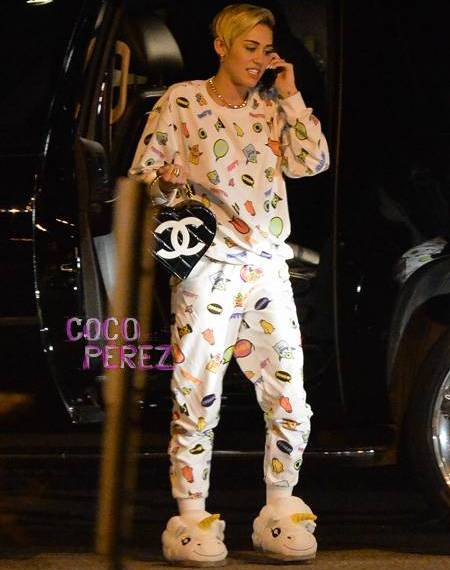In this vibrant paparazzi photo, Miley Cyrus, the famous female singer, is captured stepping out of a black SUV. She stands centered in the image, donning a quirky and colorful matching pajama set embellished with an assortment of fruits, vegetables, circles, and balloons. This vivid outfit is paired with whimsical white unicorn slippers. Miley's hair is styled in a short, almost men's haircut, and is blonde. She accessorizes with a golden chain around her neck and carries a black heart-shaped Chanel bag, featuring the iconic white "C" logo, in her right hand. Her left hand holds a cell phone to her ear. Clearly taken by a paparazzo, the scene is further adorned by a sign with "Coco Perez" written in pink letters, making for a lively and distinct capture.